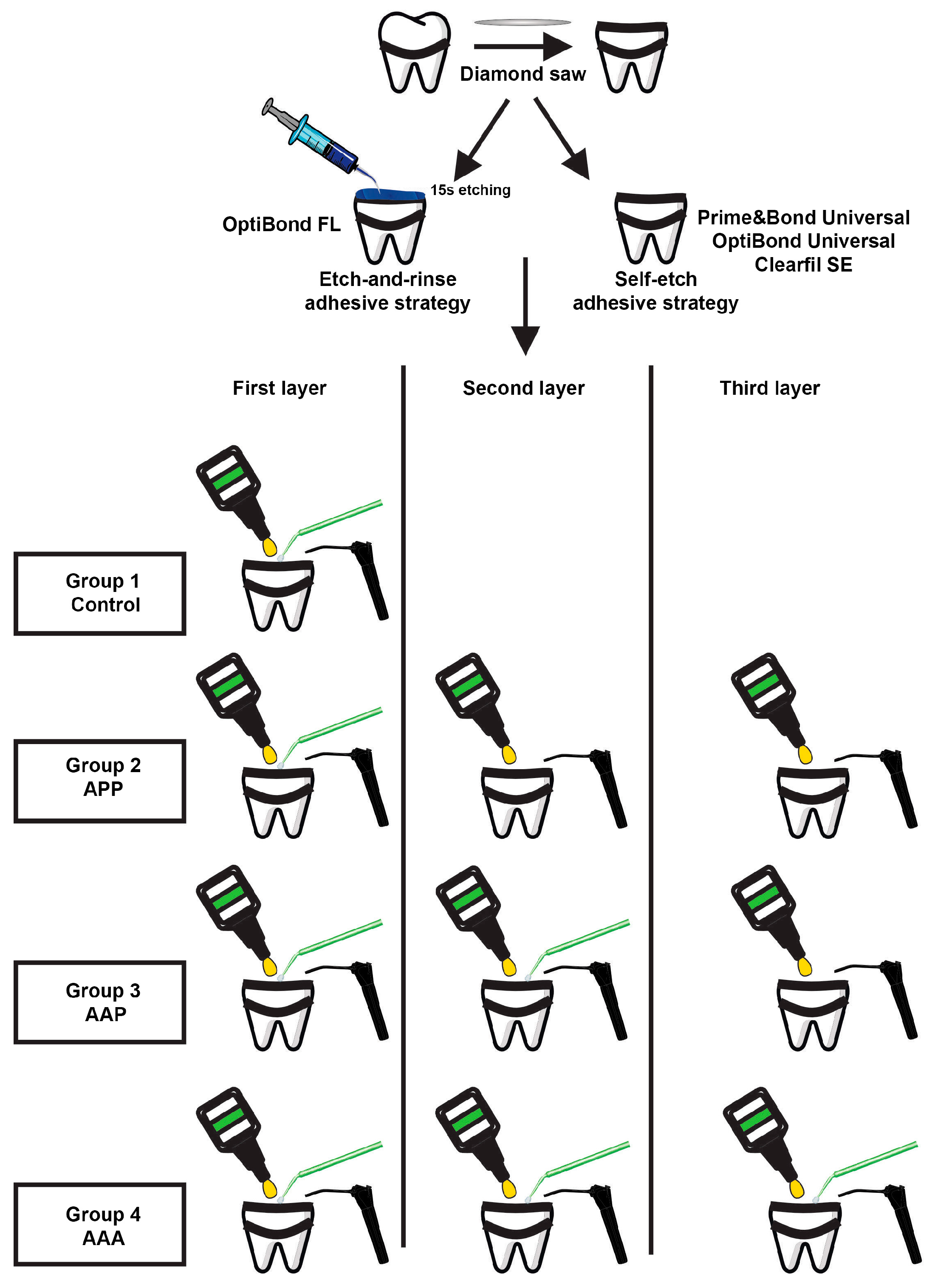The image depicts a detailed and somewhat convoluted diagram illustrating the process of bonding materials to a tooth, possibly to address cavities. The chart is segmented into three distinct layers and outlines various adhesive strategies. At the top, there's mention of a "diamond saw," likely indicating the cutting of the tooth's surface. Below this, the diagram details the application of different adhesives, including OptiBond FL, OptiBond Universal, Prime and Bond Universal, and ClearFill SE, with arrows indicating sequential steps. The second and third layers involve further adhesive applications, represented by a bottle dripping liquid onto the tooth. Various groupings are shown, labeled as control group 1, group 2 (TAP), group 3 (AAP), and group 4 (AAA), suggesting different methods or conditions used in an experimental setup. The diagram appears to aim at explaining the layering process and the specific adhesives used at each stage, likely in the context of a study on dental bonding techniques.